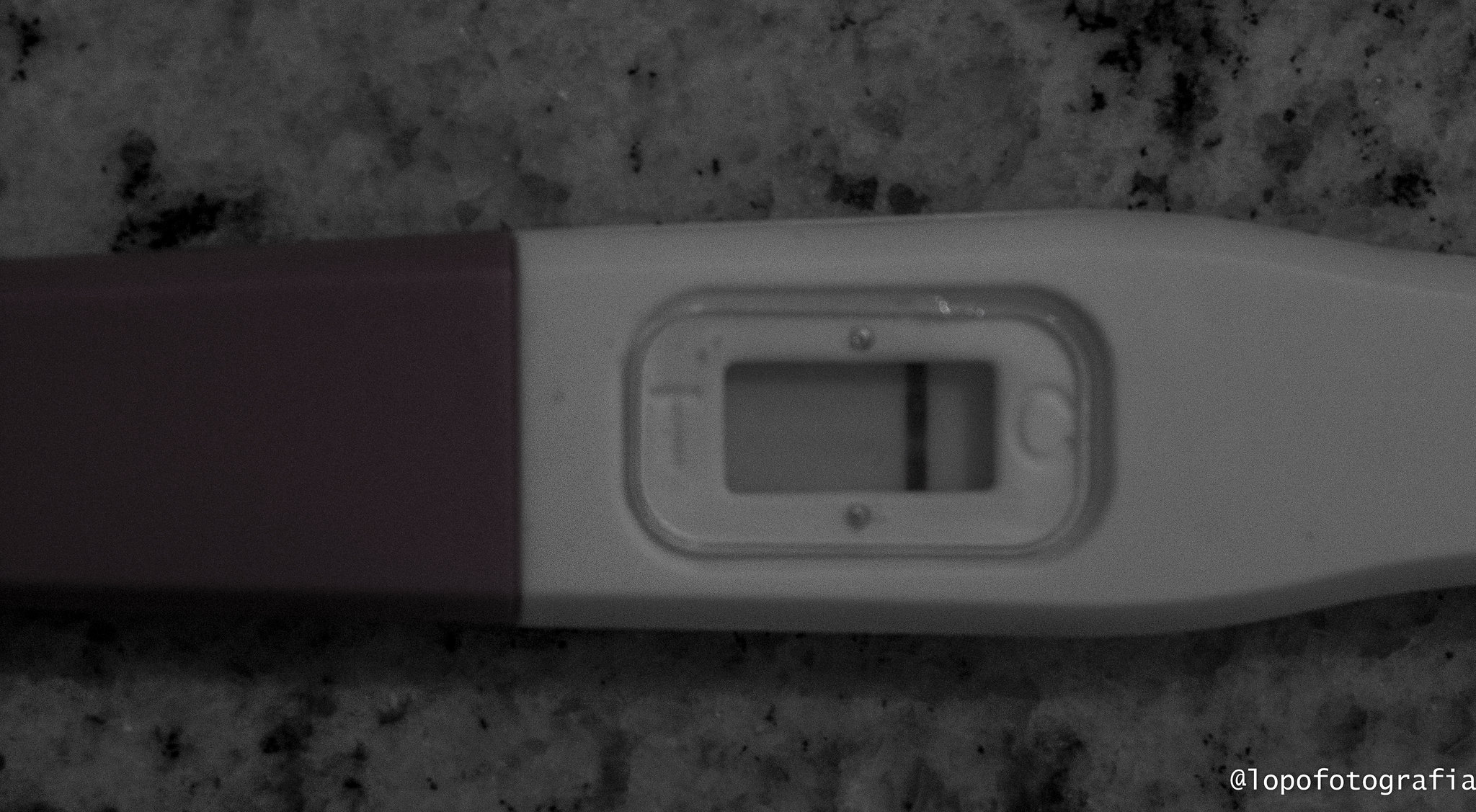A detailed image description:

The photograph displays a marble countertop with a rectangular-shaped object placed on it, which tapers slightly towards the bottom. Centered on the marble surface is an LCD screen featuring a gray background, with the letters "T" on the left side and "C" on the right side. A distinct, straight line appears on the right-hand side of the screen, adjacent to the "C." The left side of the object, near the "T," is colored red or burgundy. This object closely resembles a pregnancy test. The visible line near the "C" suggests a positive result for pregnancy. Notably, there is text at the bottom right of the image that reads "@Lopofotografia." Congratulations, Lopo, on the impending addition to your family!